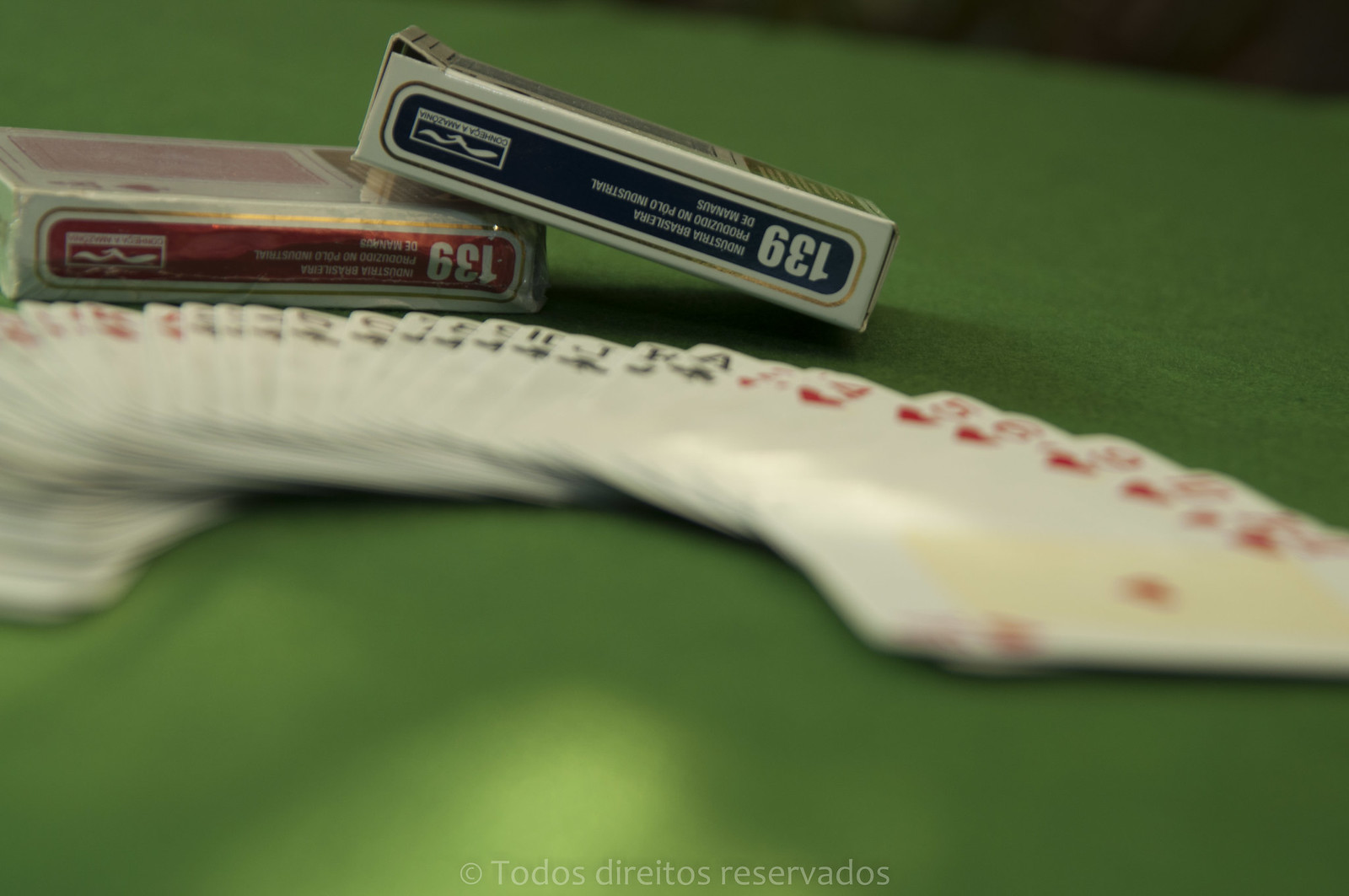A detailed caption for the image could be:

"On a green felt card table, a hand of playing cards is fanned out from left to right in the foreground, although the numbers on the cards are blurred. The card on the far right is a heart, followed by clubs. Just above this fanned arrangement are two decks of cards: a red deck lies flat on the table, while a blue deck rests on top of the red one, slightly to the right. Both decks feature the number '139' on their sides, indicating the manufacturer's mark, commonly found on professional poker or casino cards. At the very bottom of the image, a copyright notice in Spanish reads 'TOTOS, Doritos, Reservados.'"